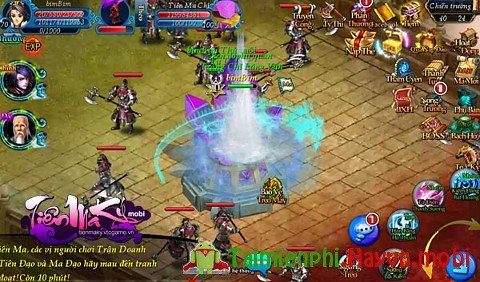In this image, a screenshot from a video game is depicted. The bottom right corner features a website link, reading "tamynvi.hayvin.mobi," accompanied by a small green Android logo. Dominating the center of the screen is a radiant, powerful flower emitting blue energy. The right side of the screen showcases various icons, including a map, inventory, and other game elements. On the left side, different playable characters are displayed, while their corresponding health bars are visible in the top left corner of the screen.